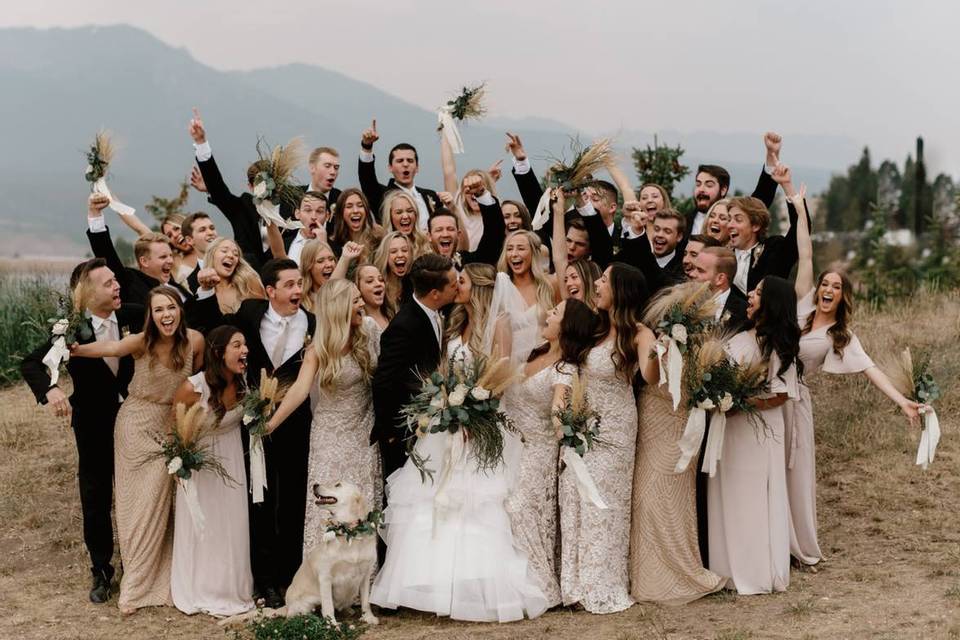In this vibrant wedding photo, taken outdoors under a subdued, cloudy sky, the bride and groom share a kiss in the center of their extraordinarily large bridal party, consisting of about 20 groomsmen and as many bridesmaids, totaling approximately 60 people. The groomsmen are elegantly dressed in black suits with white shirts and ties, while the bridesmaids wear long dresses in various shades of white, off-white, and very pale tones, including a few almost mauve. The women hold bouquets of wildflowers tied with white ribbons. The joy and excitement are palpable as everyone, including the bride holding her large bouquet, raises their hands in celebration, their faces lit up with big smiles.

An adorable golden Labrador retriever stands next to the bride and groom at the forefront, adorned with a wreath around its neck. The group stands on a patch of brown, burned-out grass in a scenic area, with a high mountain range fading into the misty background. To the right, a line of trees and bushes appears, while to the left, there's a glimpse of a river or lake. The setting, which some describe as desert-like with dirt underfoot and sparse desert plants, adds a unique charm to this joyous moment. The groom is also seen kissing a young girl, possibly a relative, as everyone in the party laughs and enjoys the heartfelt scene.